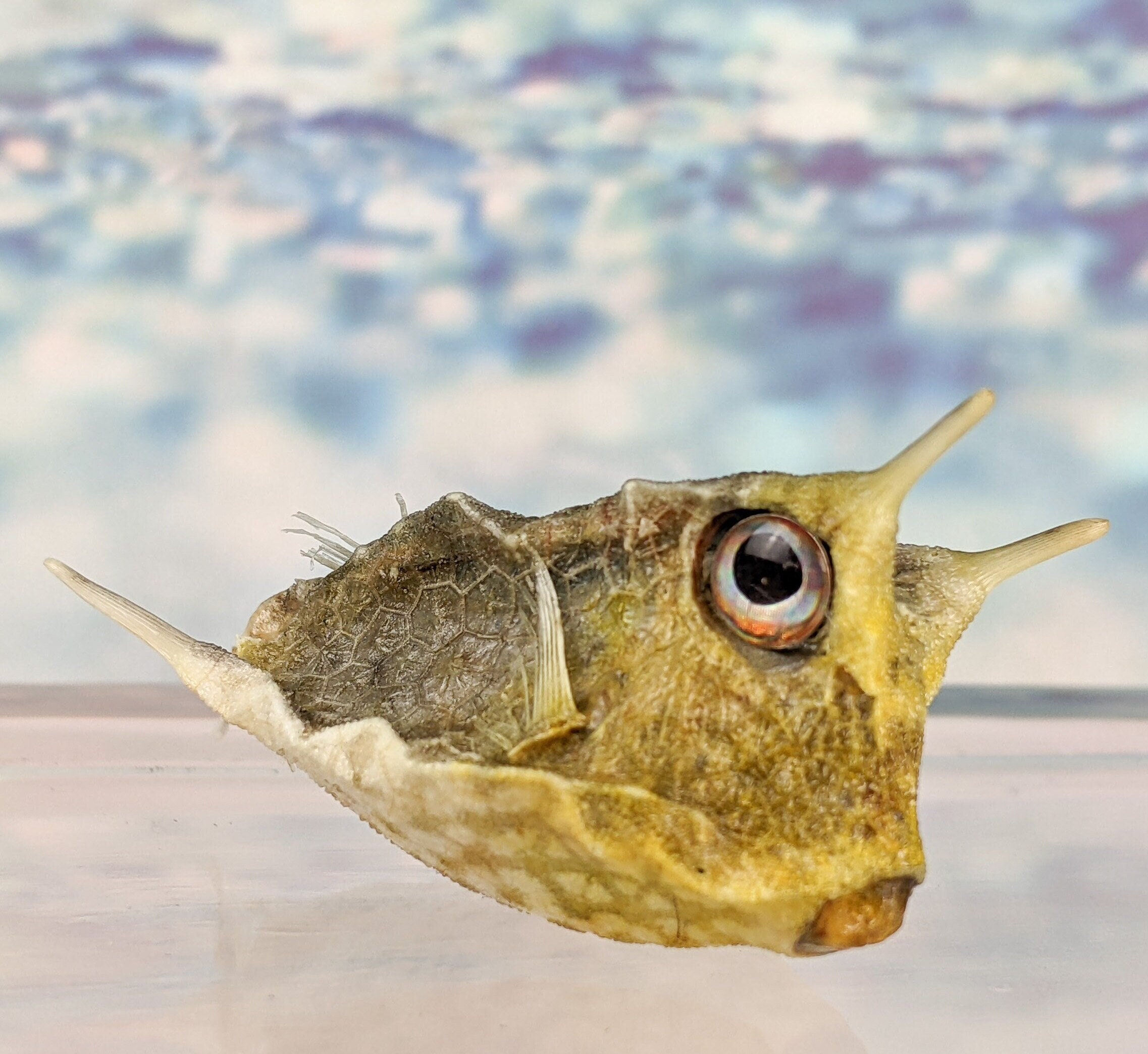This is a digitally altered and artistically manipulated photograph of an unusual sea creature resembling a fish head encased in a crab shell. The creature's triangular body sports a yellowish, leathery texture with peeling scales on the left side. Dominating the head is a single large blue eye, set against a brownish backdrop. The fish's face points to the right, slightly tilted, displaying a unique mouth with two protruding peaks or sticks at the bottom. From the top of its head, two long, straight, horn-like structures emerge, angled to the right. The background accentuates its surreal nature, blending a mottled sandy terrain below with a dark gray ocean meeting a sky painted in dreamy pink, blue, and purple hues. The creature appears almost as if it is flying or hovering over the ocean, adding to the ethereal and obviously digitally manipulated essence of the image.